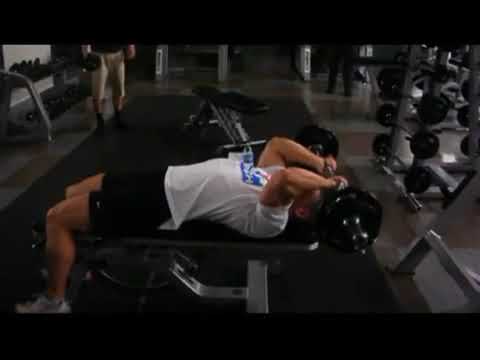In a dimly lit gym with a linoleum surface and safety mats beneath the lifting areas, a man is captured in the midst of an intense workout. Laying back on a bench, he is performing a press, his arms fully extended upwards, gripping a barbell with black iron weights. He is dressed in black shorts and a white short-sleeved t-shirt adorned with a blue design on the front. His feet are positioned towards the left side of the image, while his head and arms stretch off to the right. In the background, a man wearing shorts and possibly a black shirt watches intently, holding a dumbbell in his right hand. Racks filled with various weights and bars line the perimeter of the gym, and the photograph hints at another pair of legs or potential gym equipment further back. The image measures approximately four and a half inches by four inches.